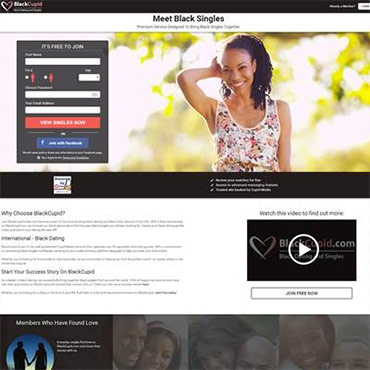This image is a screenshot with a square-like format. The upper section features a black stripe extending from the top left to the top right, containing what seems to be the BlackCupid logo on the upper right side. Below this stripe, there is another stripe with white text centered within it, stating "Meet Black Singles," accompanied by some gray text underneath that is not legible.

The entire background of the image is dominated by a photograph of a younger, dark-skinned woman with black hair. She has her right hand raised near her right ear and is wearing a floral summer shirt with a scoop neck that reveals her shoulders and arms. The backdrop consists of blurred green and white summery leaves with a lot of sunlight filtering through.

To the left of this photograph, there is a form set against a black background. The form indicates that it is free to join and includes several fields to fill in. There is a prominent red button, likely labeled "Join Now," as well as a blue button for signing in with Facebook.

On the right side of the image, there is a large, black placeholder resembling a video thumbnail, accompanied by a white button underneath that reads "Join Free Now."

The bottom section of the image contains what appear to be more images, though specific details are not clear.

Overall, this seems to be a sign-up page for the "Meet Black Singles" dating site, featuring vibrant visuals and multiple call-to-action buttons to encourage users to join.